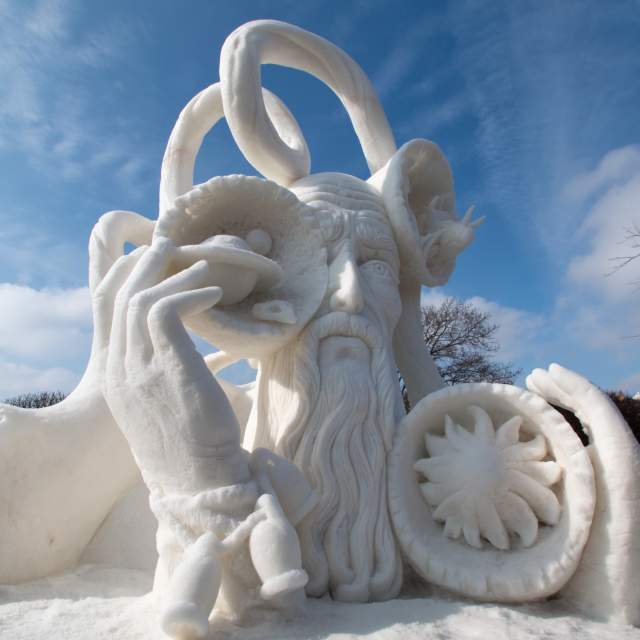In this intricate scene, the central focus is a majestic statue of a man, skillfully carved with striking detail. The statue's most distinguishing feature is its extraordinarily long beard, which cascades down and makes contact with the snowy ground below. This impressive head-and-beard sculpture exudes a sense of timeless wisdom and grandeur.

To the right of this central figure, a sculpted hand emerges, with its fingers gracefully curving to the left. Just left of this hand, there's an intriguing circular object reminiscent of a flower's bloom, its petals meticulously detailed.

On the left side of the image, another hand is depicted, its four fingers gently resting on a circular object that intriguingly encases what appears to be a UFO.

Above this enchanting scene, a looping line weaves twice before connecting to the right ear of the statue, adding an element of visual intrigue and fluidity.

The background features the serene tops of several trees, their silhouettes creating a tranquil contrast against the expansive, mostly blue sky adorned with drifting white clouds. This blend of artistic sculpture and tranquil natural elements crafts a striking and evocative visual narrative.